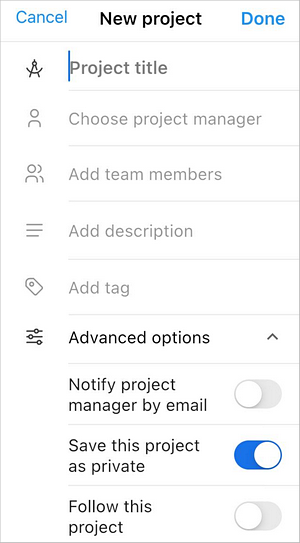The image shows a white background featuring a user interface for creating a new project. The top part includes a blue "Cancel" button and a blue "New Project" button. Below these, a "Project Title" field is highlighted with a blue cursor. There's an option to "Choose Project Manager" in gray text. Additional sections in gray include fields to "Add Team Members," "Add Description," and "Add Tag." An "Advanced Options" section is displayed in black text. To the right, there's an upward arrow, indicating an option to notify the project manager by email. Below that, a toggle bar is set to 'off'. Another toggle bar titled "Save this project as private" is switched 'on'. Lastly, there is an option to "Save or follow this project" with its toggle bar set to 'off'.